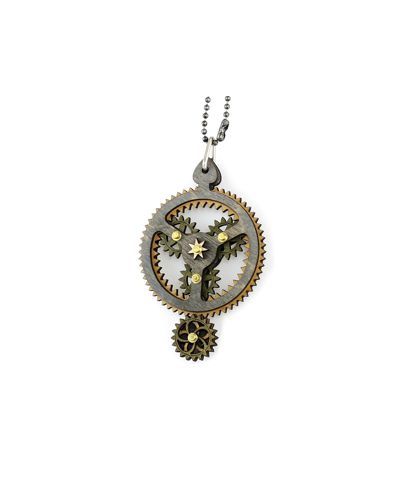This image showcases an intricately designed necklace, prominently featuring a large wooden gear as its centerpiece. The large gear is laser-cut from brown wood with varying tones and is assembled using brass hardware. Within the main gear, there are three smaller gears that closely resemble the bottom gear, showcasing fine detailing in coppery gold hues. The large gear has a metallic star-shaped piece at its center. The small gear at the bottom is accented with a green hinge linking it to the metal framework. Moreover, the top gear is silver, secured together with tiny gold screws, and there is a protruding feature with a hole through which a silver loop is threaded. This loop connects to a ball chain, hinting at its use as either a piece of steampunk-inspired jewelry or an art piece. The background is minimalistic, drawing full attention to the detailed assembly and craftsmanship of the gear necklace.